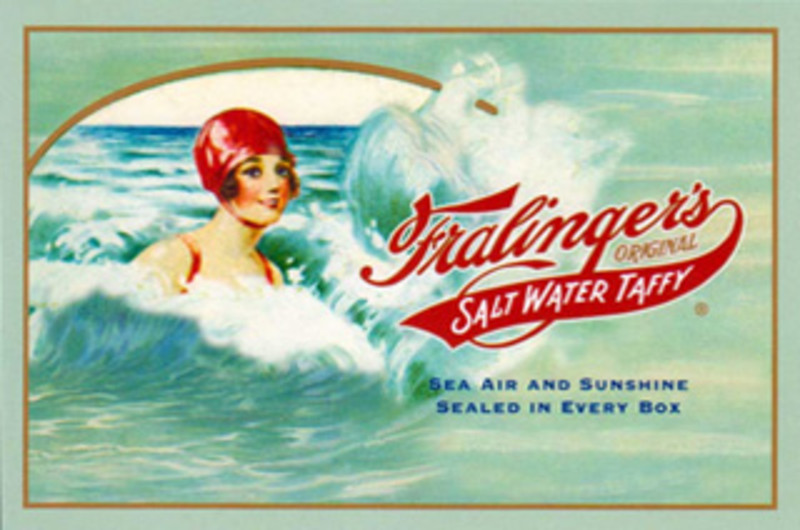This vintage advertisement, seemingly from the 1920s, promotes Fralinger's original saltwater taffy. The ad features a vivid scene of the ocean with a woman in a red bathing cap and matching bathing suit, emerging from teal and blue crashing waves. The background comprises a blend of sky and sea, creating a refreshing and nostalgic ambiance. The ad is framed by a tan rectangle with gold trim and a curved line, adding to its old-fashioned charm. Prominently displayed on the right side, red lettering spells out "Fralinger's original," followed by a red banner with white text reading "saltwater taffy." Below, in blue letters, it states "sea air and sunshine sealed in every box," capturing the essence of the seaside treat. The overall aesthetics are marked by a light blue hue, with the framing and decorative elements underscored in gold, evoking a sense of timeless appeal.